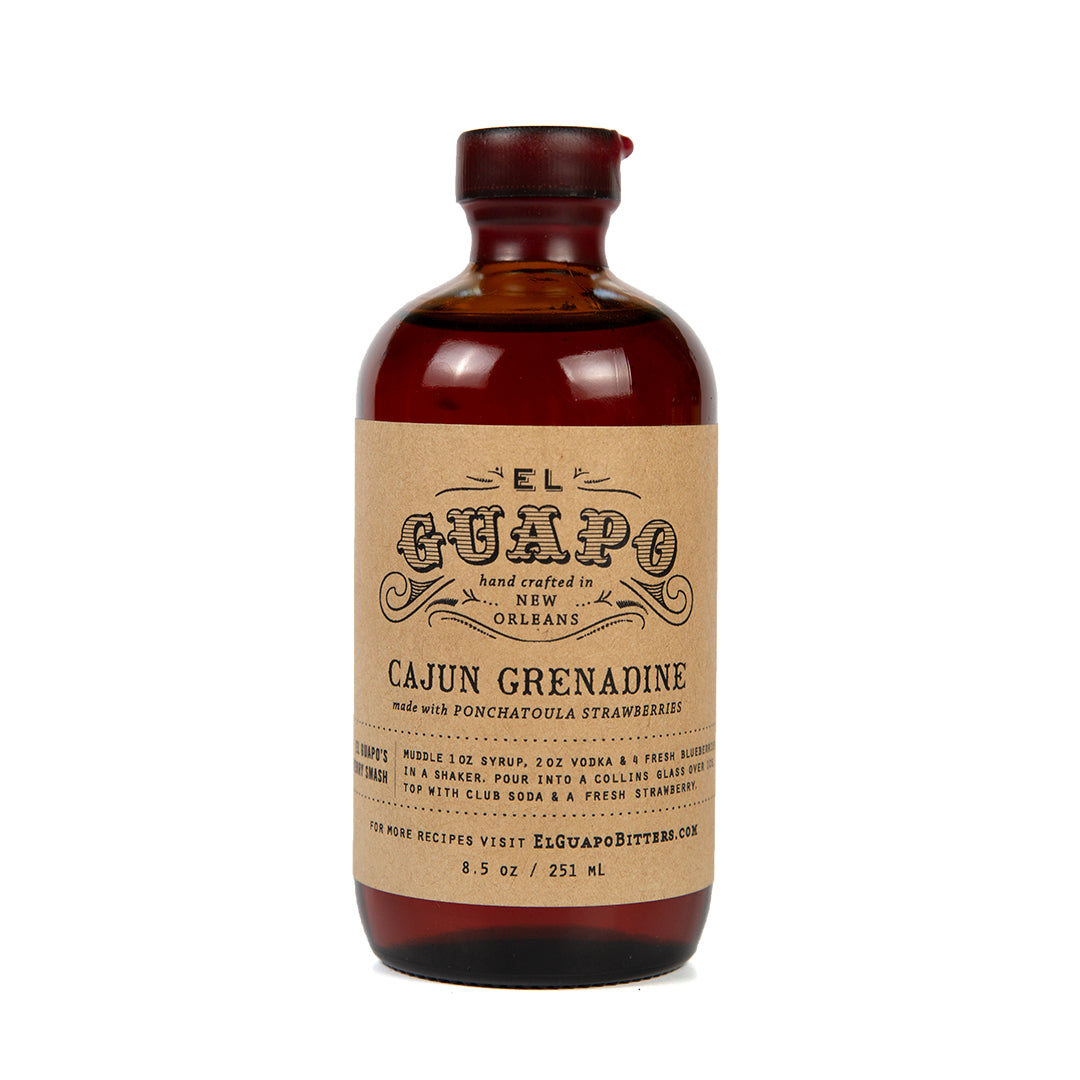This image showcases a short, stocky bottle of El Guapo Cajun Grenadine, prominently placed against a plain white background with no visible borders. The dark red bottle, which appears to be either glass or plastic and about four inches high, has a sealed cap in the same rich hue. The bottle's neck narrows before widening slightly where a cork might fit. A sizable, light brown paper label adorns the bottle's front, bearing a stylized, old-timey black text that reads "El Guapo," followed by "handcrafted in New Orleans." Ornamental illustrations surround the text, enhancing the vintage aesthetic.

Below the main header, the label continues with "Cajun Grenadine," in larger letters, and specifies "made with Ponchatoula strawberries." Further down, a cocktail recipe is printed, although it is somewhat difficult to read. It details instructions to "muddle 1 oz. syrup, 2 oz. vodka, and 4 fresh blueberries in a shaker," then "pour into a Collins glass over ice," and "top with club soda and a fresh strawberry." The label also directs viewers to "for more recipes visit ElGuapoBitters.com." At the very bottom, the bottle's volumetric capacity is noted as "8.5 ounces / 251 milliliters."